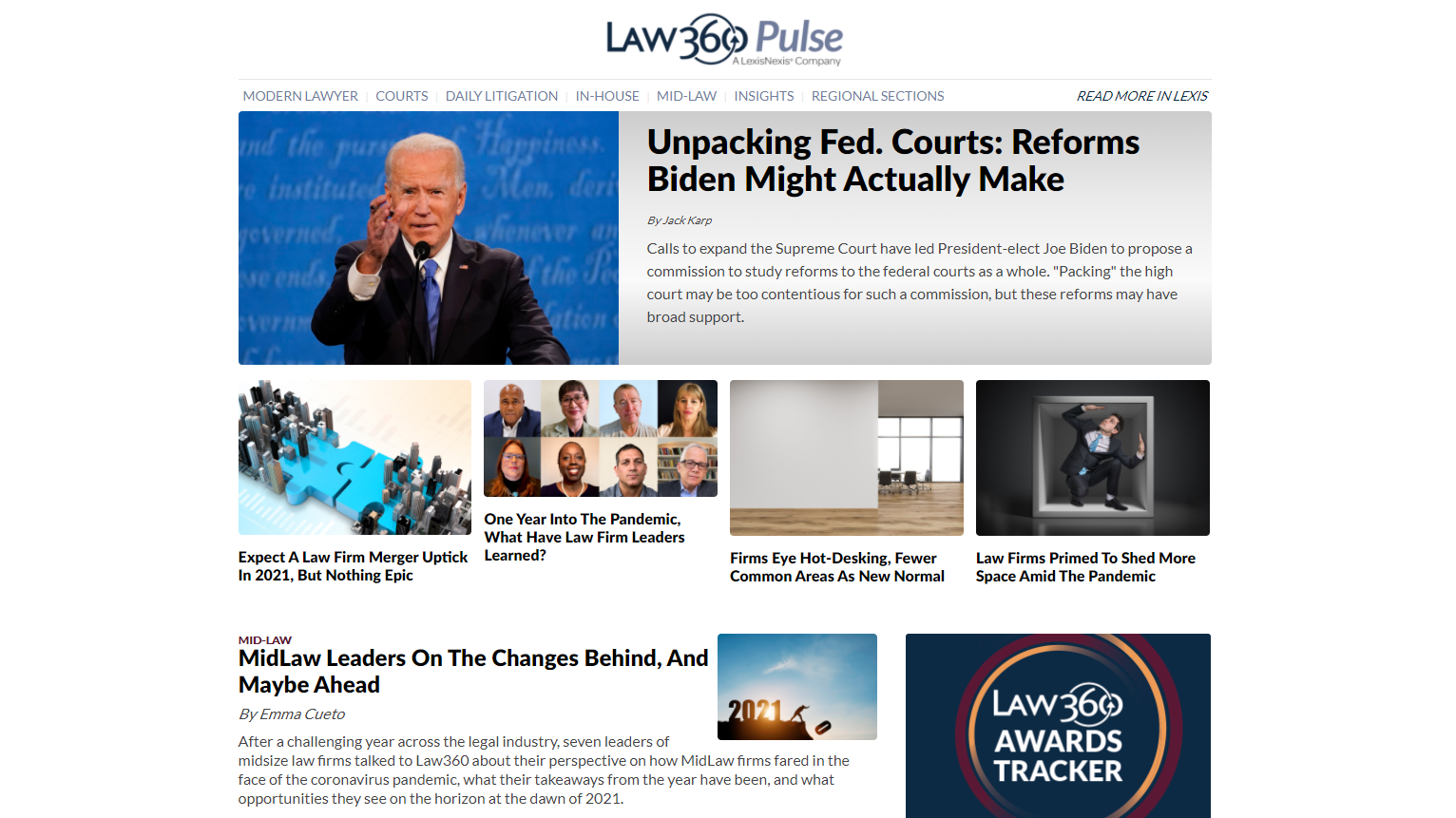The image is from a page titled "Law 360 Pulse," prominently displayed at the top. The "Law 360" logo features a unique design where the numbers "3" and "0" are circled, encompassing the number "6," all set in a dark blue or black color, with the word "Pulse" in gray.

Below the title, there are several tab headings, including "Modern Lawyer," "Courts," "Daily Litigation," "In-House," "Mid-Law," "Insights," and "Regional Sections." There is also a heading labeled "Read More," which appears to direct to Lexis.

The page features multiple images and headlines:
1. **Joe Biden Image:** President Joe Biden poses against a blue background wearing a black suit. The headline reads, "Unpacking Fed Courts: Reforms Biden Might Actually Make." Below this are four lines of black text, which are too small to be legible.
   
2. **Puzzle Pieces Image:** Two blue puzzle pieces are shown fitting together. Below it, the caption states, "Expect a Law Firm Merger Uptick in 2021 but Nothing Epic."

3. **Law Firm Leaders Image:** This image features eight different people. The caption reads, "One Year Into the Pandemic, What Have Law Firm Leaders Learned?"

4. **Large Room Image:** Depicts a spacious room with white walls, a brown wooden floor, windows, and some chairs. The caption under this image says, "Firms Eye Hot Desking, Fewer Common Areas as New Normal."

5. **Male in Suit Image:** A man in a suit is shown standing next to a box. The caption reads, "Law Firms Primed to Shed More Space Amid the Pandemic. Mid-Law Leaders on the Changes Behind and Maybe Ahead."

6. **2021 Image:** Shows the year "2021," with a figure pushing the zero off. 

In the lower right corner of the page, within a blue rectangle, it says "Law 360 Awards Tracker."